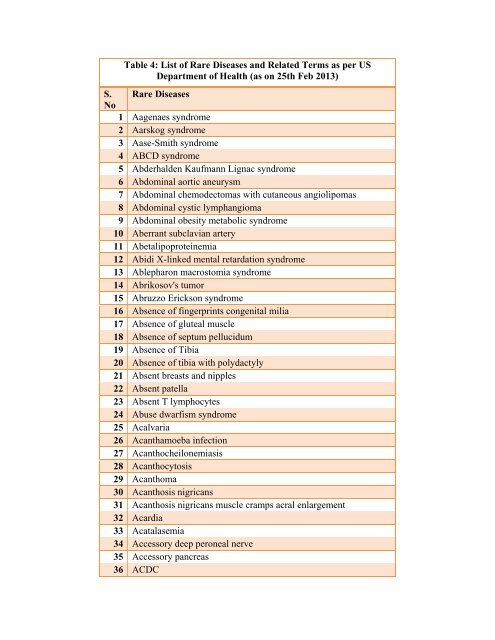The image is a detailed portrait-oriented chart titled "Table 4, List of Rare Diseases and Related Terms as per U.S. Department of Health, as on 25th February, 2013." The chart is structured into two columns: a narrow left column labeled "S. NO" listing numbers 1 through 36 in bold, and a main column labeled "Rare Diseases." The diseases are presented in alphabetical order, each row alternating between white and cream-colored backgrounds. The rare diseases listed include Aagenaes Syndrome, Aarskog Syndrome, and extend through to various other conditions such as ABCD Syndrome, Abdominal Obesity Metabolic Syndrome, and Abrikosov's Tumor. The title of the chart and the column headers are in bold black text, providing a clear and organized presentation of 36 rare diseases.